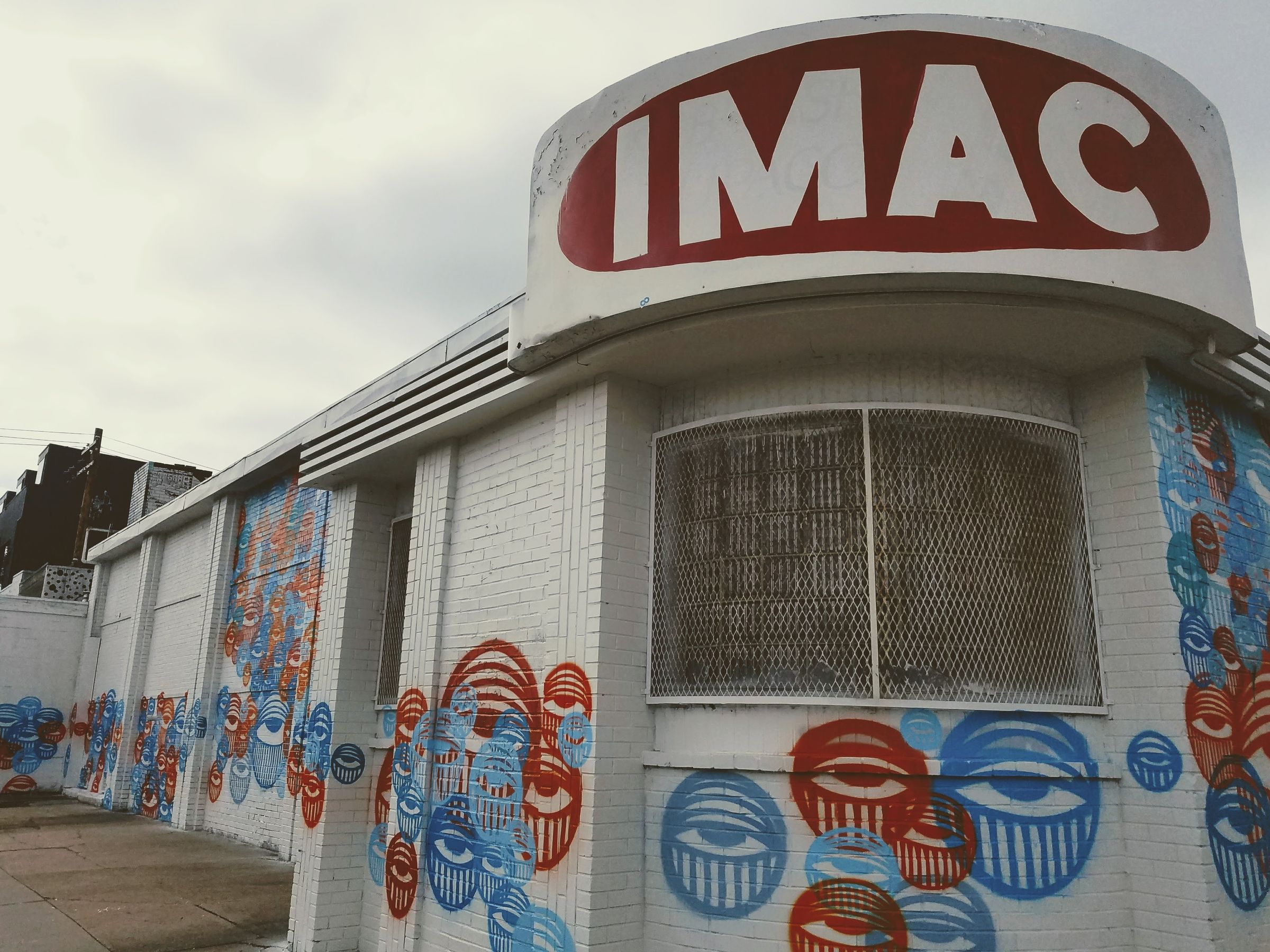This outdoor photograph captures a primarily white-brick building against an overcast sky filled with light and darker gray clouds. The main focus is on the building, which prominently features the word "IMAC" in white letters on a dark red oval sign at the top. The bricks are uniformly painted white, and the windows are protected with metal grating. Below the sign, repetitive graffiti decorates the walls: a design of overlapping eyes in red and blue colors. Each eye is barely open, with vertical lines descending from them, creating a pattern that covers nearly every visible section of the building's façade. The sidewalk in the bottom left corner is gray, and another structure with a black and white rooftop, alongside a brown post, is visible in the far back left of the image.